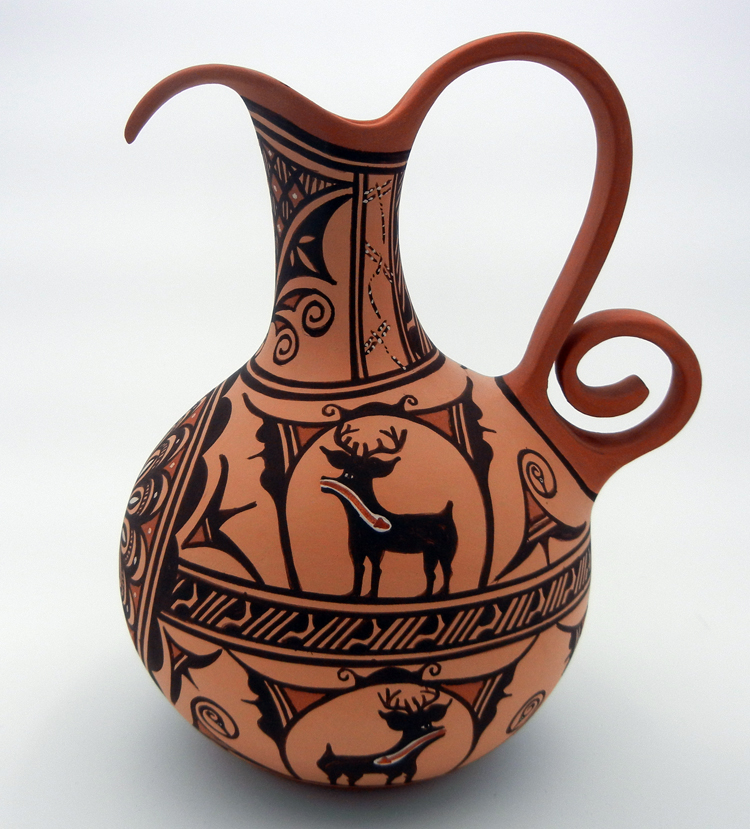This intricately designed piece of pottery is a vase characterized by its curvy, swirling form with a thin neck that expands into a round, bulbous bottom. The vase features a mix of colors, primarily a brownish-copper base with contrasting lighter and darker brown accents, especially around the handle and the top where the spout is located. The elaborate handle, which swirls at the base like a curly pig's tail, adds to its ornate appearance. 

Black and gray patterns adorn the neck, and below it, the central section of the vase showcases a detailed depiction of a horned and hoofed animal, likely a species resembling a deer, elk, or reindeer, complete with large horns. An arrow runs through the mouth and down into the stomach of this animal, which is surrounded by intricate, banner-shaped patterns and positioned under an archway. Another similar animal appears below it, set within the same decorative framework. The pot is further embellished with abstract patterns, lines, and floral decorations, enhancing its already elaborate design. The overall effect is one of complex artistry and detailed craftsmanship, with a striking combination of detailed patterns and vivid imagery.